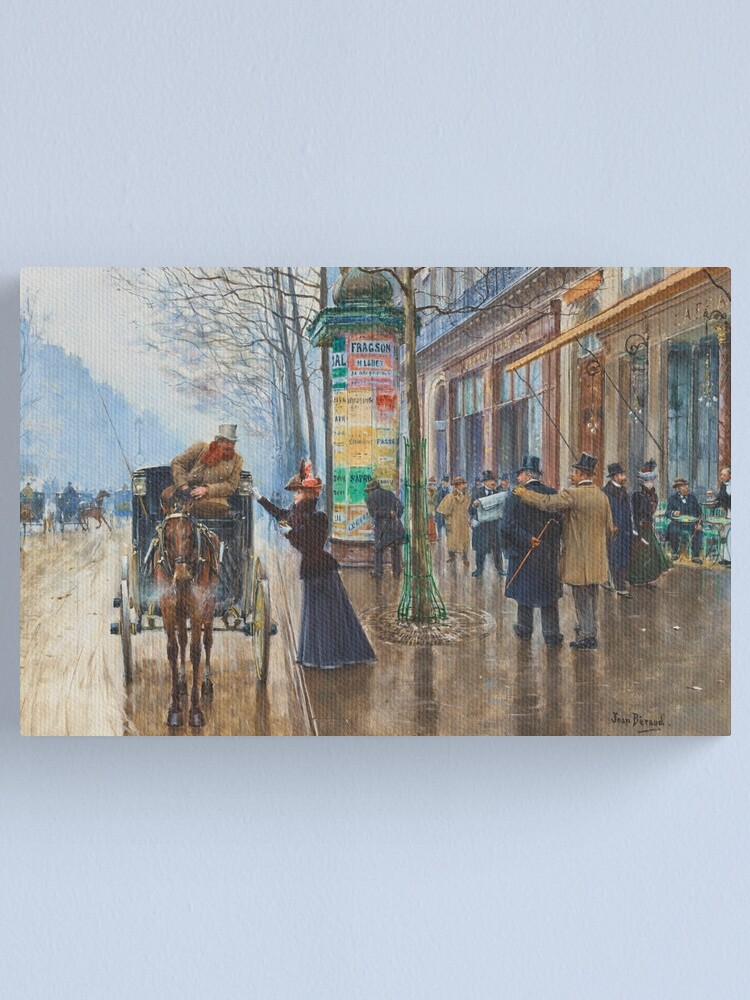The painting, created by Jean Barad, depicts an 18th-century city street bustling with activity. The scene features a row of shops lining a broad sidewalk where men and women stroll, all dressed in period attire with top hats, long skirts, and canes. In the center of the image, a woman wearing a long skirt, black top, and a reddish hat is engaged in conversation with a coach driver. The coach, pulled by a single horse, boasts four large wheels. The driver is distinguished by his top hat, red scarf, and tan jacket. 

The setting suggests a winter atmosphere, indicated by the barren trees in the background. Across the street, additional coaches and buggies move along, adding to the vibrancy of the scene. A marquee sign hangs at the edge of the sidewalk, though its text is too fine to discern. Notably, a man stands on the sidewalk engrossed in a newspaper, further enriching the historical ambiance of the scene. The painting, rendered in full color and with a canvas-like texture, hangs on a light blue or gray wall, with Barad's signature visible in the bottom right corner.